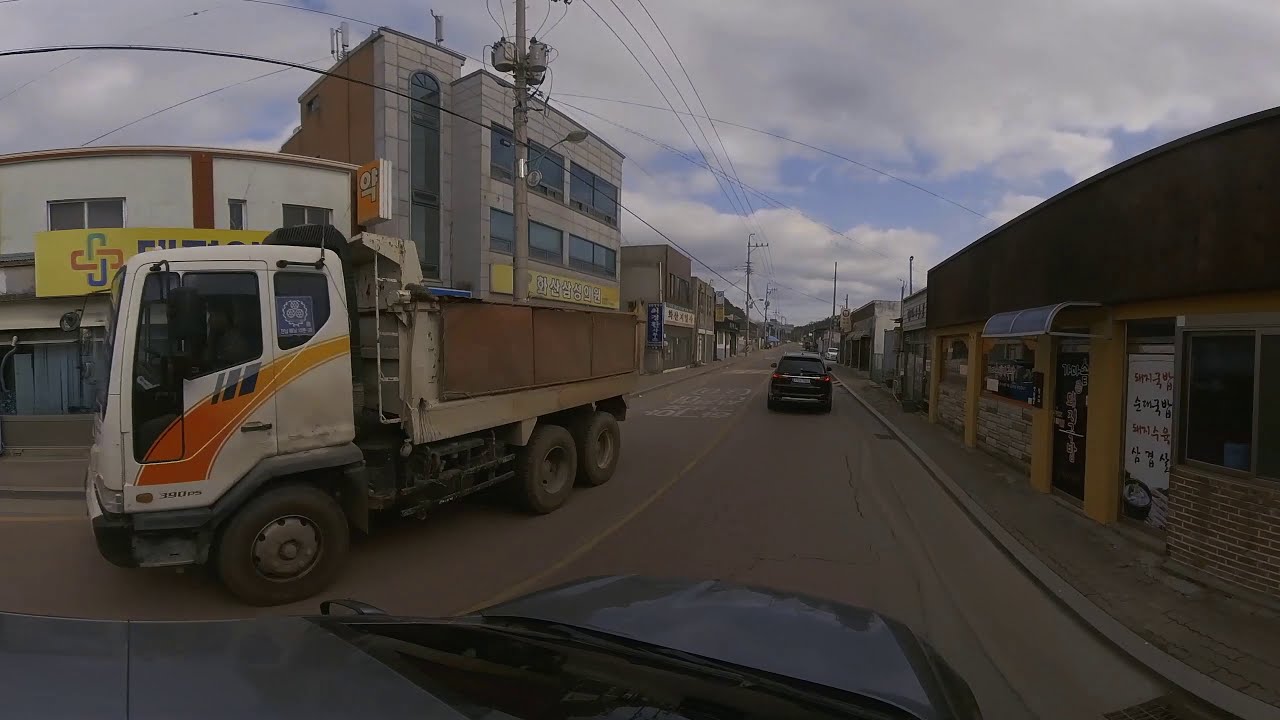This daytime photograph, taken from the first-person perspective of a gray SUV's dash cam, captures a bustling city street in Korea. The scene features cracked asphalt of an old foundation and spans two lanes, with one heading forward and the other in the opposite direction. Immediately ahead, a white car is parked by the curb, and another SUV is seen driving. To the left side of the SUV, a white and orange dump truck carries an empty load. The street is flanked by commercial buildings, some of which display Korean or Japanese writing and have glass doors beneath metal awnings. Storefronts line both sides of the street, with sidewalks and curbs clearly visible. Power lines with transformers stretch across the sky, which is predominantly cloudy but with patches of blue. The street appears quiet, devoid of pedestrians, and features white lettering painted on the road.